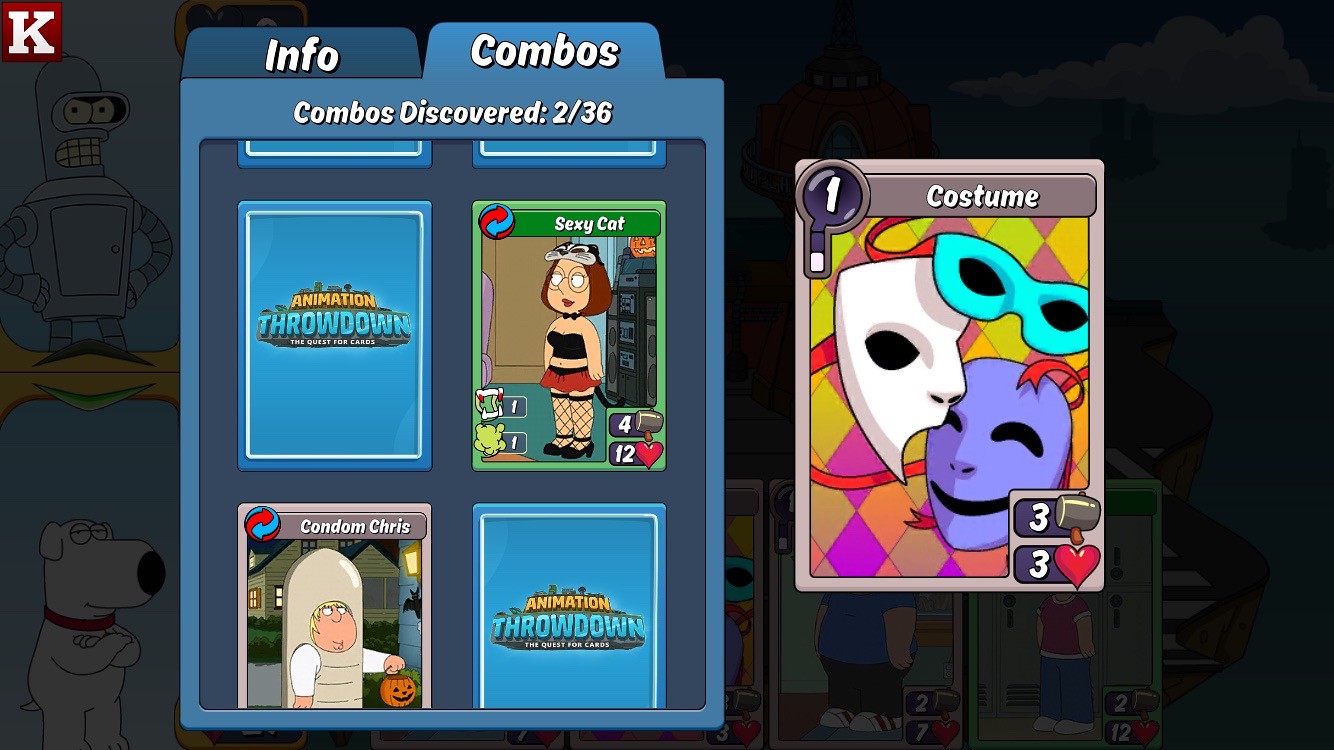The image appears to be a screenshot from a Family Guy-themed mobile card game. The background is predominantly black, featuring a prominent blue box with two tabs at the top: "Info" (left, dark blue) and "Combos" (right, lighter blue). The "Combos" tab is selected, displaying the text "Combos discovered: 236". Below the tabs, there are four cards arranged in two rows on the left side of the screen. At the top left is the back of a card labeled "Animation Throwdown". To its right is another card titled "Sexy Cat", depicting Meg Griffin in a bustier top, short skirt, and fishnet stockings. The bottom left card is "Condom Chris", showing Chris Griffin dressed in a condom costume holding a pumpkin, implying trick-or-treating. The bottom right card is another "Animation Throwdown" card displaying its back. To the right of these four main cards is a smaller card titled "Costume", featuring theater masks and an eye mask. It also shows a "1" in the top corner, a "3" with a hammer in the bottom left, and a "3" with a heart in the bottom right. In the upper left corner of the blue box, a white "K" is seen against a red background.